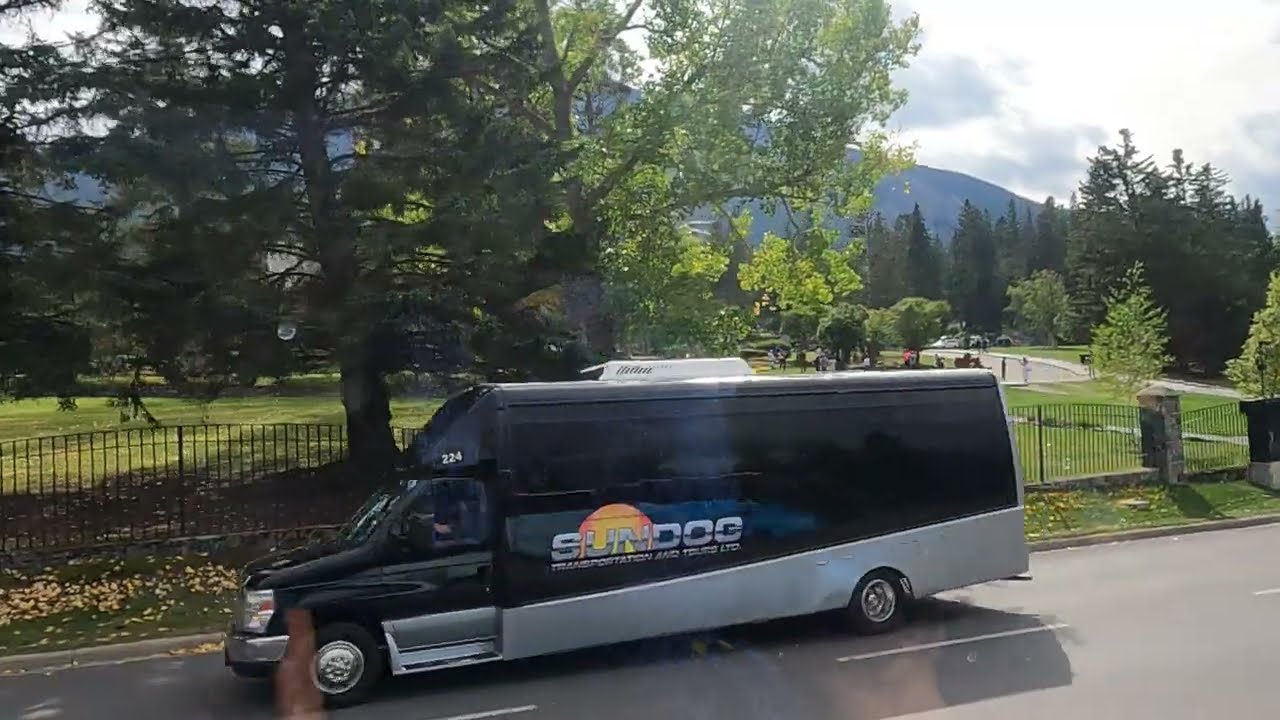In this detailed outdoor photograph taken in broad daylight, a distinctive black and gray bus labeled "Sundogs Transportation and Tours LTD" with a sun logo and the number 224 on top is prominently featured. The bus, which has a unique longer front end and a white fan covering on top, is parked on a road. The setting appears to be in front of a serene park area enclosed by grills and walls, teeming with greenery and numerous pine trees. Way off in the distance, people can be seen, possibly taking photographs. Beyond the park area, a vast meadow stretches out, ending at a very large blue mountain under a clear sky with some scattered clouds. The scene is further enriched by the sunlight illuminating the surroundings. The photograph appears to have been taken from within another vehicle, as indicated by the faint reflection or shadow of a person in the bottom corner of the image.